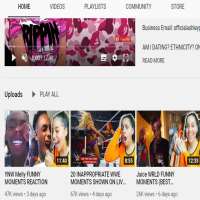This image appears to be a screenshot from a video-sharing website, displayed against a neutral (black or white) backdrop. At the top left, navigation options are listed in black font: "Home," "Videos," "Playlists," "Community," and "Store."

Below this navigation bar, there is a large video preview box. This box features a prominent white play symbol indicating that the video is ready to be played. The visual content within the video is a blend of pink, white, and maroon colors swirled together. On the left side of this preview, there is black text that seems to spell out "RIPPIN," though it's partially obscured and unclear. Similarly, black text appears on the right side of the preview but is too blurry to decipher.

Beneath this, the label "Uploads" is clearly written in black, accompanied by a play symbol and the phrase "Play All." Below these elements, there are three smaller video preview boxes arranged horizontally.

1. The first box shows three African American faces presented side-by-side, as if they are part of a collage.
2. The second box features a dark-skinned girl with dark hair, wearing an orange shirt. She is positioned in the bottom right corner of the frame and has a shocked expression.
3. The third box again showcases the same girl in the orange shirt, this time with her hair pulled back. She is smiling and located in the right-hand side of the frame.